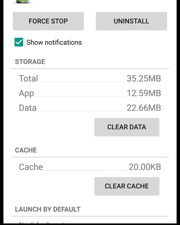The image depicts a memory usage report for a software program, formatted within a rectangular frame. The visual dimensions are such that the length of the left and right sides are twice that of the top and bottom sides. Notably, portions of the top and bottom sections of this report are missing from view. Surrounding the report on the left, right, and bottom sides is a thick black border, while the top side remains borderless.

At the very top of the image, there are two adjacent gray rectangles, each containing black text in all capital letters. The left rectangle displays "FORCE STOP," and the right rectangle shows "UNINSTALL." Directly below the "FORCE STOP" rectangle, the text reads "SHOW NOTIFICATIONS" beside a checkbox that is currently checked, indicated by a green box containing a white checkmark.

The background for the remaining portion of the report is white, contrasting with the gray text. The memory usage details are organized in a chart format, listing:

- Total: 35.25 MB
- App: 12.59 MB
- Data: 22.66 MB

Further down, towards the right, there's another gray rectangle with black text in all capitals that reads "CLEAR DATA."